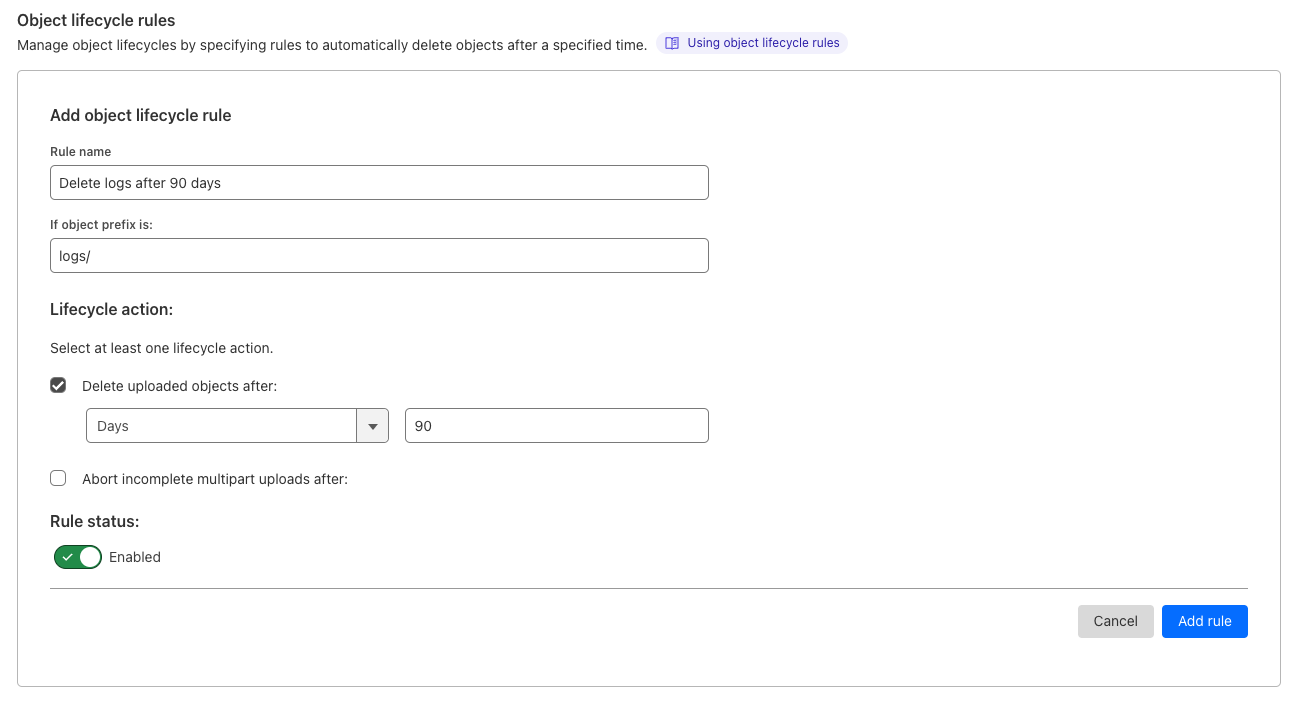Screen capture showcasing a configuration interface with a white background and black text focused on managing object life cycles. At the top, the header reads "Object Life Cycle Rules" with a subtext explaining that these rules allow automatic deletion of objects after a specified period.

Just below, in a blueish-purple hue, the header "Using Object Life Cycle Rules" is prominently featured. The central part of the image displays a large white box bordered by a thin gray line, containing a form titled "Add Object Life Cycle Rule" in black text.

The form includes several fields:
- "Rule Name" accompanied by a white input box containing the text "Delete logs after 90 days."
- "If object prefix is" followed by an input box with "log/" already filled in.
- "Life Cycle Action" urging the user to select at least one action. Below this, a gray checkbox is marked against "Delete uploaded objects after" with an adjacent input box pre-filled with "90" days.

Another section reads "Abort incomplete multi-part uploads after" but no time frame is specified in the available text box.

The rule's status is listed as "Enabled," denoted by a green box with a white circle. To conclude the form, there are two buttons at the bottom: a gray "Cancel" button and a blue "Add Rule" button.

The image quality is crisp and clear, with no pixelation or blurring, making all elements easily distinguishable.